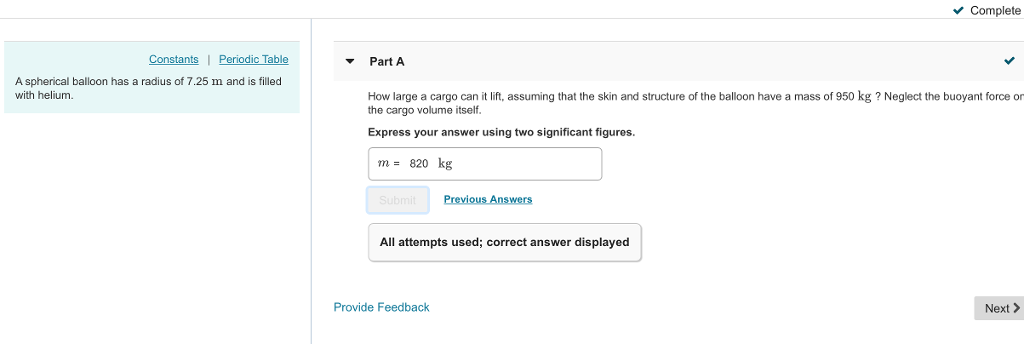### Descriptive Caption:

The image depicts a digital quiz interface, likely designed for educational purposes. The layout is characterized by a two-pane structure. On the left pane, there is a physics problem that reads, "A spherical balloon with a radius of 7.25 meters is filled with helium." To the right, there's a detailed segmented area titled "Part A," which asks, "How large a cargo can it lift?" Additional conditions include: "Assuming that the skin and structure of the balloon have a mass of 950 kilograms, neglect the buoyant force and the volume of the cargo itself. Express your answer using two significant figures."

Below the question, there is a single text field intended for inputting the computed answer. A button labeled "Previous Answers" suggests that users can review their past attempts. To aid further, a line of text hints at previous calculations with "m = 820 kilograms mass," presumably offering an initial value that needs to be used in the solution. The screenshot indicates that users may have encountered difficulties with this problem, as noted with the phrase "All attempts use correct answer displayed," implying multiple attempts and corrections.